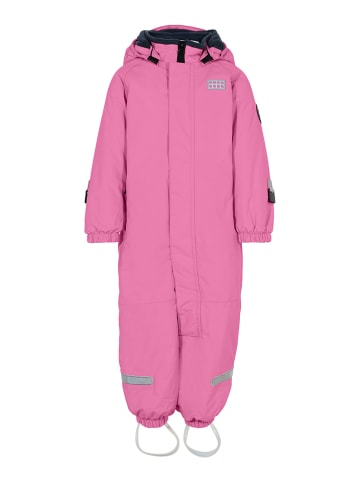In this image, there is a children’s snowsuit displayed against a completely white background, emphasizing its details vividly. The snowsuit is a medium shade of pink with a hood that's folded back. The hood's neck lining is black, adding contrast to the overall pink garment. The front of the snowsuit features a zipper that is fully covered by a pink fabric flap, giving it a sleek appearance. On the upper right side (viewer's perspective) of the chest, there is a gray rectangular patch decorated with white lines forming a grid pattern. The sleeves end in elastic cuffs, and the lower legs also feature gray rectangular accents. Uniquely, the ankles have clear, white elastic loops, reminiscent of stirrups, that would help keep the snowsuit in place over footwear. This image, likely destined for an online store or catalog, is focused solely on the snowsuit, making it the central and sole subject in the frame.